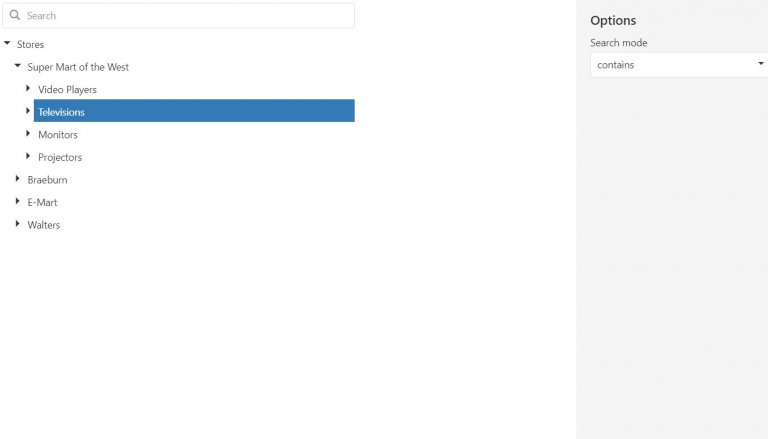A detailed and polished caption for the described screenshot would be:

"Screenshot of a website's search page with a white background. The page is divided into two main sections. On the left side, there is a search box labeled 'Search' accompanied by a magnifying glass icon. Below the search box, there's an expanded drop-down menu. At the top of this menu, the heading 'Stores' is visible. The menu appears open with 'Supermart of the West' selected. Additional categories under 'Supermart of the West' are listed: 'Video Players,' 'Televisions,' 'Monitors,' and 'Projectors,' with 'Televisions' highlighted by a blue box indicating it has been clicked. Also listed are 'Braeburn,' 'Emart,' and 'Walters,' aligned with 'Supermart of the West' on the left margin. To the right, there's a gray rectangular section titled 'Options, Search Mode,' featuring a white box labeled 'Contains' with a dropdown menu beside it."